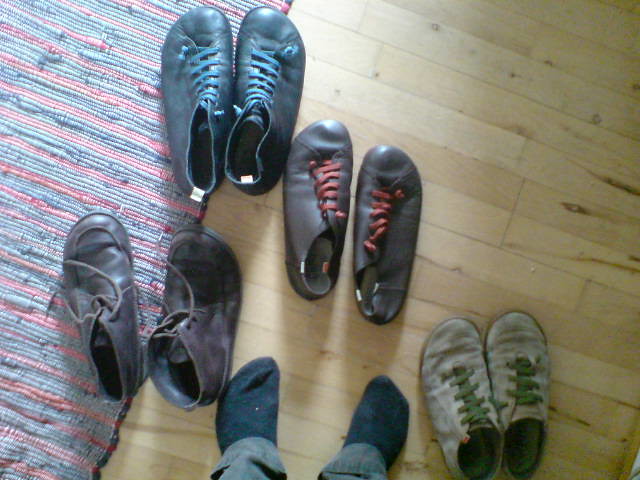This image, captured from approximately five feet above, depicts a person standing in front of four pairs of somewhat tattered, differently colored men's shoes on a light hardwood floor. The shot is taken looking straight down. The bottom of the image displays their legs clad in green pants and feet in black socks. 

The hardwood floor, composed of thin, long planks, spans the right side of the image. A rug with blue and red stripes covers the left side. Positioned among the shoes, from left to right, are:

1. A pair of high-ankle brown leather boots with untied brown laces, which appear worn-in.
2. Black shoes with blue laces located at the top left of the frame.
3. Low-ankle brown shoes with red laces situated directly in front of the observer's feet.
4. Tan-colored shoes with green laces on the right side of the frame, also low-ankle.

Sunlight streams from the top of the image, suggesting the presence of a window above, enhancing the detailed contrast between the hardwood floor and the striped rug.